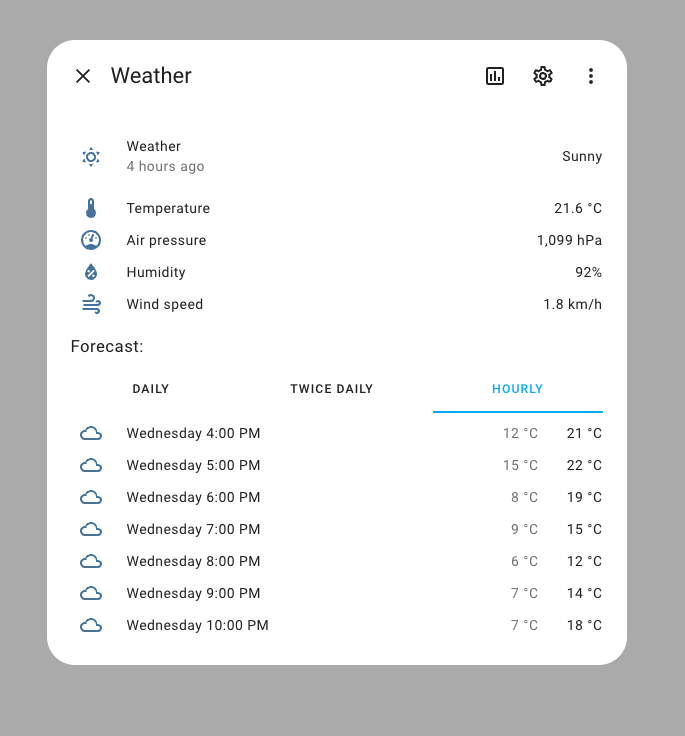**Detailed Weather App Interface Description**

The image displays a weather application interface, seemingly from a mobile device, showing detailed weather information. At the very top of the interface, the bold title "Weather" is prominently displayed. Adjacent to this title on the right side, there is a chart icon, a settings gear icon, and a menu represented by three vertical dots.

Below the main title, the word "Weather" appears again, this time in smaller text, accompanied by the note that the data was updated "4 hours ago." Each weather metric presented in the interface is accompanied by a corresponding icon to the left. These icons include a sun for current conditions, a thermometer for temperature, a barometer for air pressure, a droplet for humidity, and a wind vane for wind speed.

The weather conditions reflect sunny skies with a reported temperature of 21.6 degrees Celsius. The air pressure is listed as 1,099 hPa, though the relevance of this figure might be unclear to some users. Humidity levels are notably high at 92%, described as "hot" and "thick." The wind speed is relatively low at 1.8 kilometers per hour.

Beneath this weather summary, there is a section labeled "Forecast." This section features columns for different forecast intervals: daily, twice daily, and hourly, with the "Hourly" tab currently highlighted in blue. Detailed hourly forecasts for Wednesday are provided, starting from 4 p.m. with 12 degrees Celsius and a high of 21 degrees Celsius. Subsequent hourly readings include:

- 5 p.m.: 22 degrees Celsius
- 6 p.m.: 19 degrees Celsius
- Following hours indicate a temperature decrease down to 12 degrees Celsius before rising back up to 14 and 18 degrees Celsius by 9 p.m.

The entire interface is bordered by a gray frame, providing a clean and structured layout for the weather information.